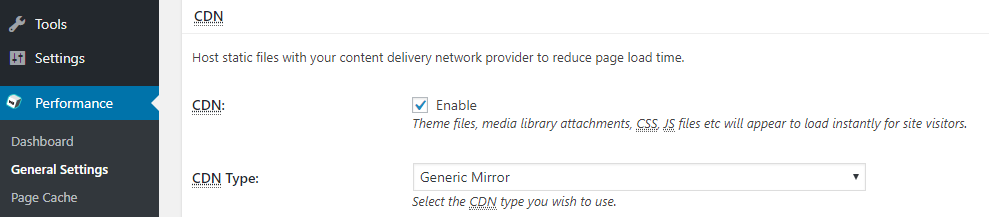The image depicts a digital interface with a focus on website performance optimization. On the left-hand side of the screen, there is a narrow, black, vertical panel featuring various menu options listed in a column: "Tools," "Settings," "Performance," "Dashboard," "General Settings," and "Page Cache." The "Performance" option is highlighted in blue with an arrow pointing inward, while "General Settings" is displayed in brighter colors, suggesting it is currently selected.

Occupying the majority—approximately 80%—of the right-hand side of the screen, there is a detailed section labeled "CDN." Below this title, a horizontal divider line separates the main content, which reads: "Host static files with your content delivery network provider to reduce page load time." Another line below reiterates "CDN," accompanied by a checkbox labeled "Enable." This checkbox is marked to indicate it is active. 

Further details specify that enabling the CDN will make "theme files, media library attachments, CSS, JS files, etc., appear to load instantly for site visitors." Additional options include "CDN type," which is set to "generic mirror." A drop-down menu is present to select the CDN type, although the available choices are not visible in the image.